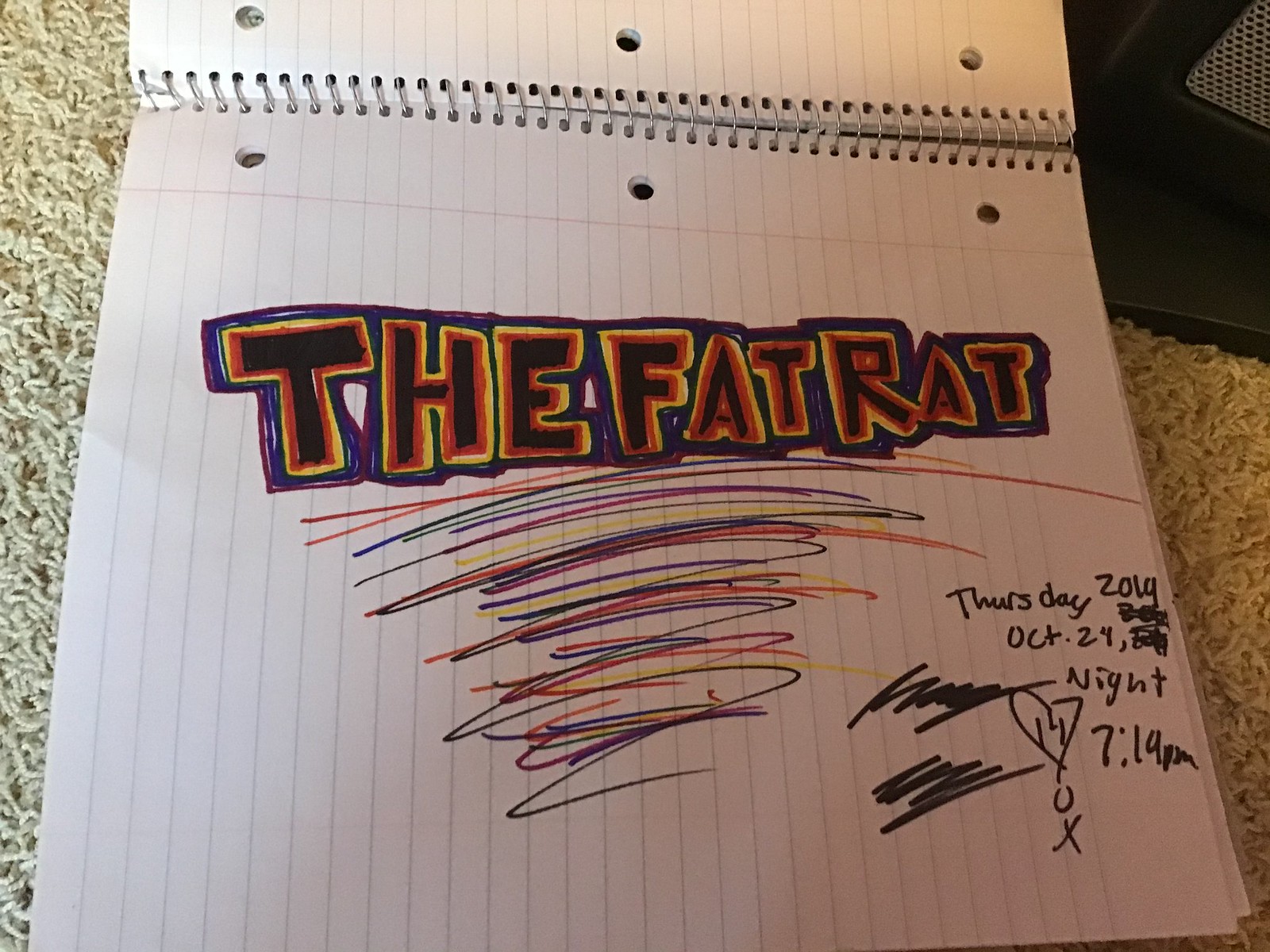This is a landscape-oriented drawing on spiral notebook paper, directly attached to the notebook. The artwork features a blue outline framing the central text. The text itself reads "The Fat Rat" in a mix of orange, yellow, and black letters, with the spaces between the letters filled in black. Below the main title, there's an array of colorful scribbles in red, purple, yellow, and black. In the lower left-hand corner, the text "Thursday 2014, October 24th" is written in black, followed by a time notation, "night 7:14 p.m." Nearby, a heart symbol, the number zero, and an 'x' are also scribbled in black ink.